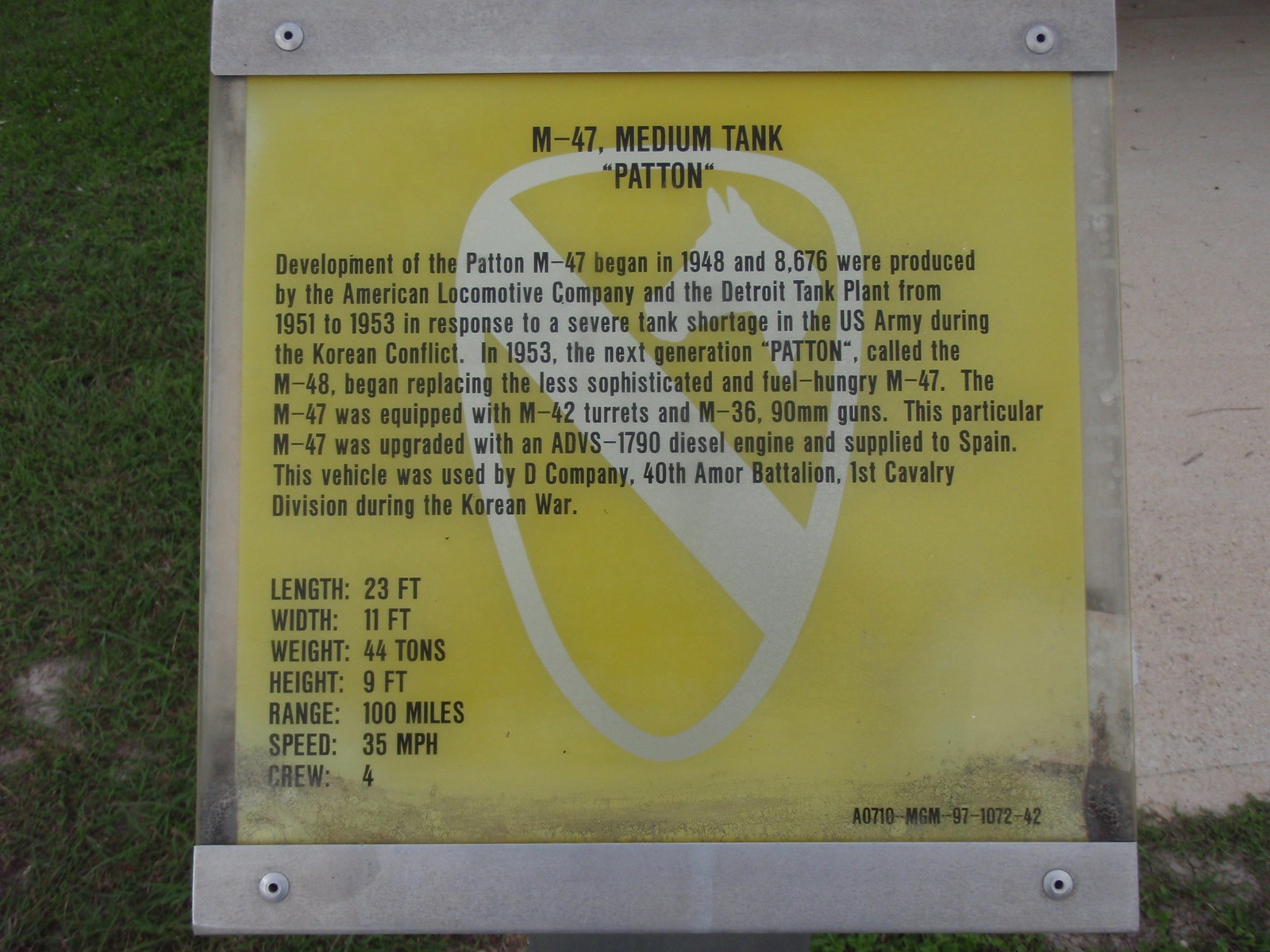The photograph captures an outdoor information plaque set against a backdrop of green grass on the left and a tan rock on the right. The plaque rests on the ground and features a transparent yellow sheet secured by metal bars at the top and bottom, each with screws in the corners. At the top of the plaque, in bold black font, the words "M47 Medium Tank" are prominently displayed, followed by the word "Patent." Below this title, a comprehensive block of black text provides detailed information about the M47 Medium Tank. The plaque is adorned with a white crest featuring a horse's head in the upper section. On the left side towards the bottom, a list of specifications—length, width, weight, height, range, speed, and crew—is neatly arranged in black font, each accompanied by corresponding numerical values. At the bottom right-hand corner, a string of letters and numbers is printed in small black font. The plaque provides extensive details about the tank, making it a valuable source of information for visitors.